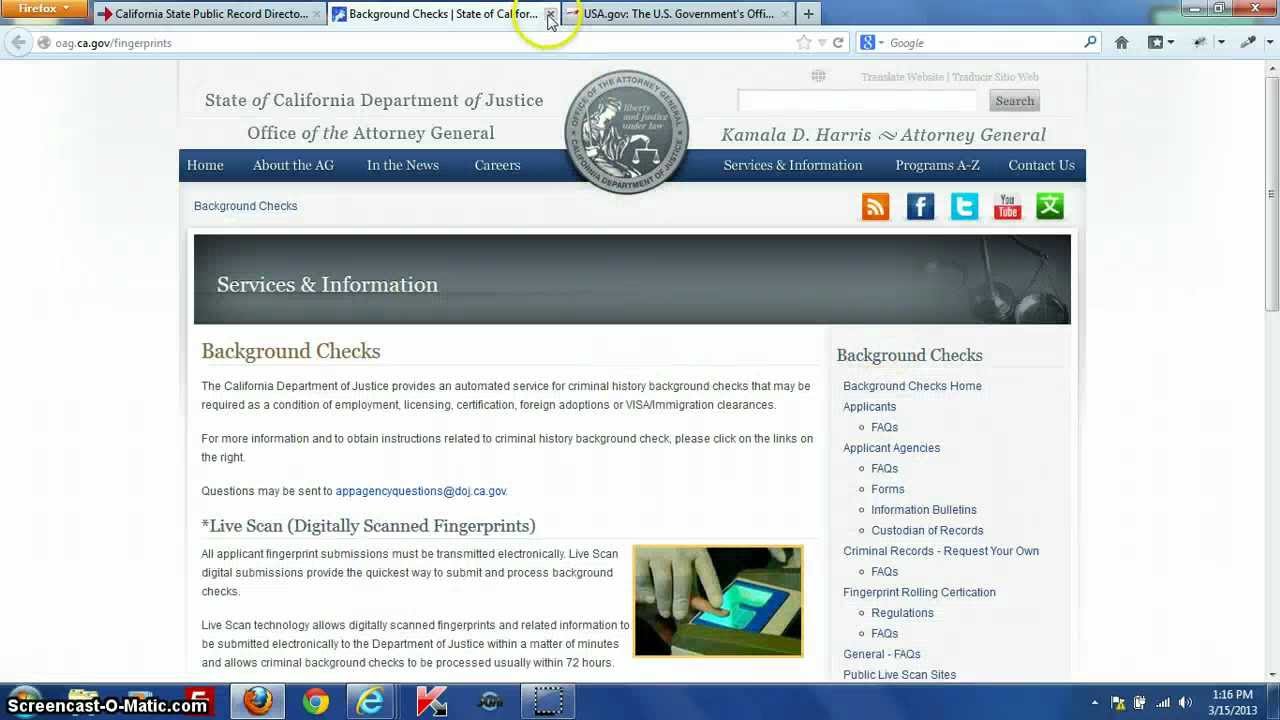This screenshot captures a detailed view of a desktop browser with multiple tabs open. The interface is shown with a yellow hue in the upper left corner. Across the top, several tabs are visible, including those for the California State Public Record Directory, Background Checks for the State of California, and USA.gov, the U.S. government's official portal. A yellow circle highlights the Background Checks State of California tab, emphasizing an arrow pointing to the "X" icon to close the tab.

The bottom portion of the screen displays the State of California Department of Justice Office of the Attorney General's website, specifically the Background Checks section. This section has a gray border with the headings "Services and Information" and "Background Checks" in a brownish color. The text explains that the California Department of Justice offers an automated service for criminal history background checks required for various purposes such as employment, licensing, certification, foreign adoptions, or visa immigration clearances.

The right side of the screen provides further navigation options within the Background Checks section, including links to Background Checks Home, Applicants, Applicant Agencies, Criminal Records, Request Your Own, Fingerprint Certification, General Facts, and Public Live Scan. This detailed layout helps users navigate through the various services related to background checks provided by the California Department of Justice.